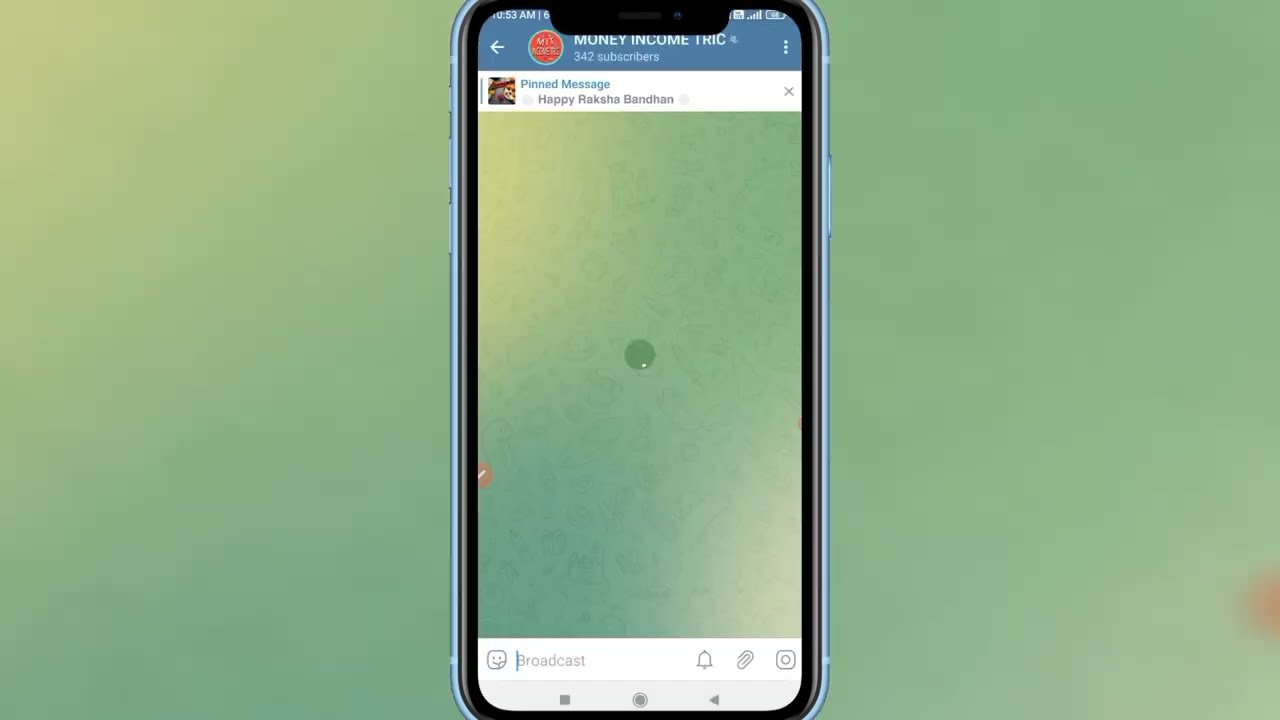In the image, a cell phone occupies the center third from top to bottom against a blurred green and yellow background. The phone, possibly an iPhone with a blue case, displays a social media or messaging app interface. At the top of the phone screen, amidst a blue header with white text, it reads "money income, 342 subscribers," followed by a white strip with a pinned message that begins with "happy R-A-K-S-H-A" and includes additional text that's difficult to decipher. The phone screen and the background share similar green and yellow hues, creating a blended visual effect. Standard phone icons such as the battery percentage, internet connection, and time appear at the top, while the bottom of the screen features typical messaging symbols like a broadcast caption, bell, paperclip, and camera icon, indicating it is a chat interface. The overall aesthetic is characterized by a predominantly green palette interspersed with blotchy, faded yellow patches.